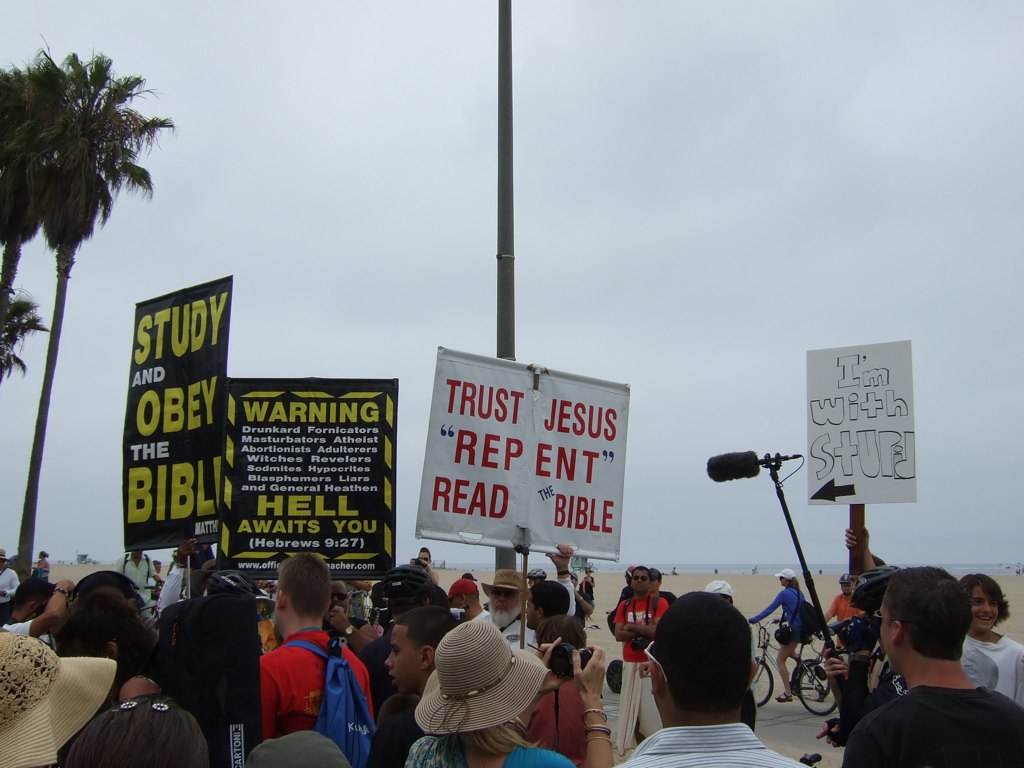In the photograph, a protest is taking place along a sandy beach with the ocean visible in the background. A group of people is prominently featured, holding various signs with religious messages. One sign, in white with bold red text, reads "Trust Jesus, Repent, Read Bible." Another sign, in black with striking yellow text, urges, "Study and Obey the Bible." Among the signs is a stark warning: "Warning, Hell Awaits You." To the right of this group, a woman stands out, holding a contrasting placard. Her sign is white and humorously states, "I'm with stupid," with an arrow pointing towards the individuals carrying the aforementioned religious signs. This scene juxtaposes serious religious campaigning with a touch of irony.